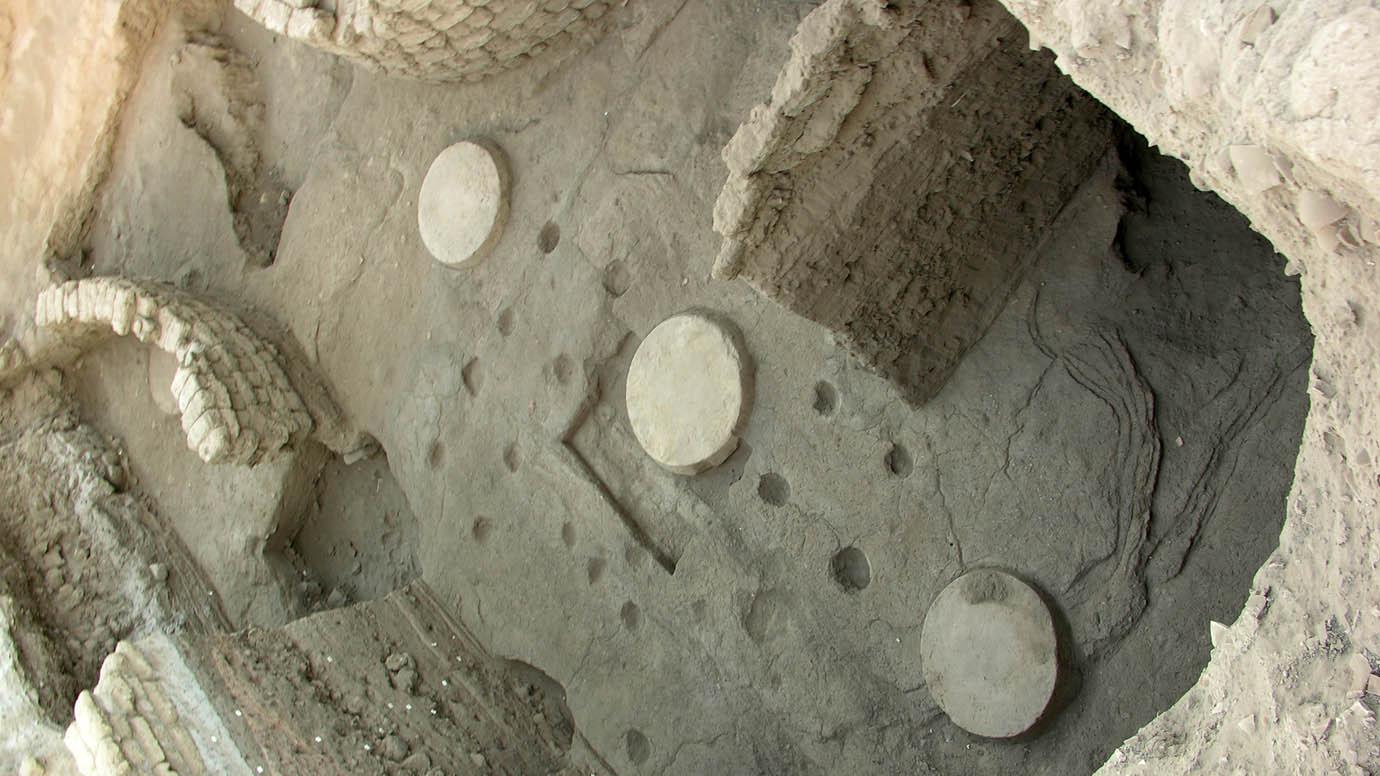The image depicts an aerial view of what appears to be an archaeological excavation site or a ruin in a desert landscape. The photograph is slightly askew, requiring a tilt to the right to view it correctly. The site is characterized by unfinished and crumbling formations of rocks, bricks, clay, and concrete materials, all in shades of gray. 

Notably, there are several roundish enclosures and small walls that give the impression of a structure that was either left incomplete or is deteriorating over time. In the bottom section of the image, positioned equidistantly from each other, are three circular discs or indentations. To the right of these discs, there is a small stone curved wall extending off the image. Below the middle disc, a rock protrusion juts out into the area, also extending out of the frame.

On the left-hand side of the image, there is a smaller, round dug-out area with an adjoining trench and a wall of mud and stone that continues off to the left. At the top of the image, you see the opposite face of the main excavation area, with another stone wall that descends to the left, ending near the top of the dug-out section.

The ground within the site has a lighter concrete color with various circular and square indentations scattered throughout, indicating either different phases of excavation or signs of structural wear and tear. The overall scene provides a glimpse into a place rich in historical significance but marred by the passage of time and the elements.